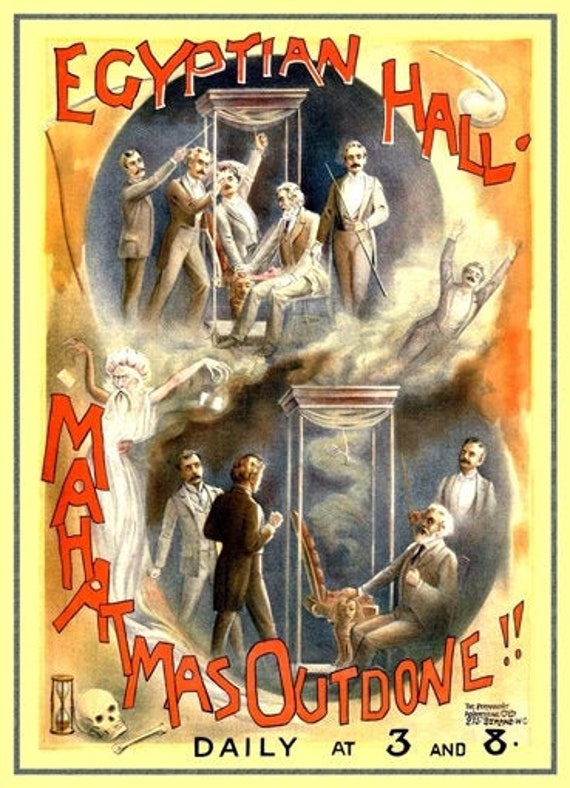This antique theatrical poster, primarily in shades of yellow and white, advertises a performance at Egyptian Hall with bold red lettering at the top stating "Egyptian Hall." The design includes a blue border around the central artwork, which features an illusion act. In the scene, four men surround a transparent box where a man appears to vanish and re-emerge as a ghostly figure. The poster's background shifts from a yellowish-orange hue to a dark navy blue or black, with intricate black-and-white drawings of the performers. Among the illustrations is a depiction of an elderly man with a long white beard and robe, striking a dramatic pose with his hands raised. At the bottom, the red text reads "Mahatma's Outdone," along with the showtimes "daily at 3 and 8." The overall sepia-toned, black-and-white thematic elements lend a timeless, early 20th-century feel to this classic magic show advertisement.